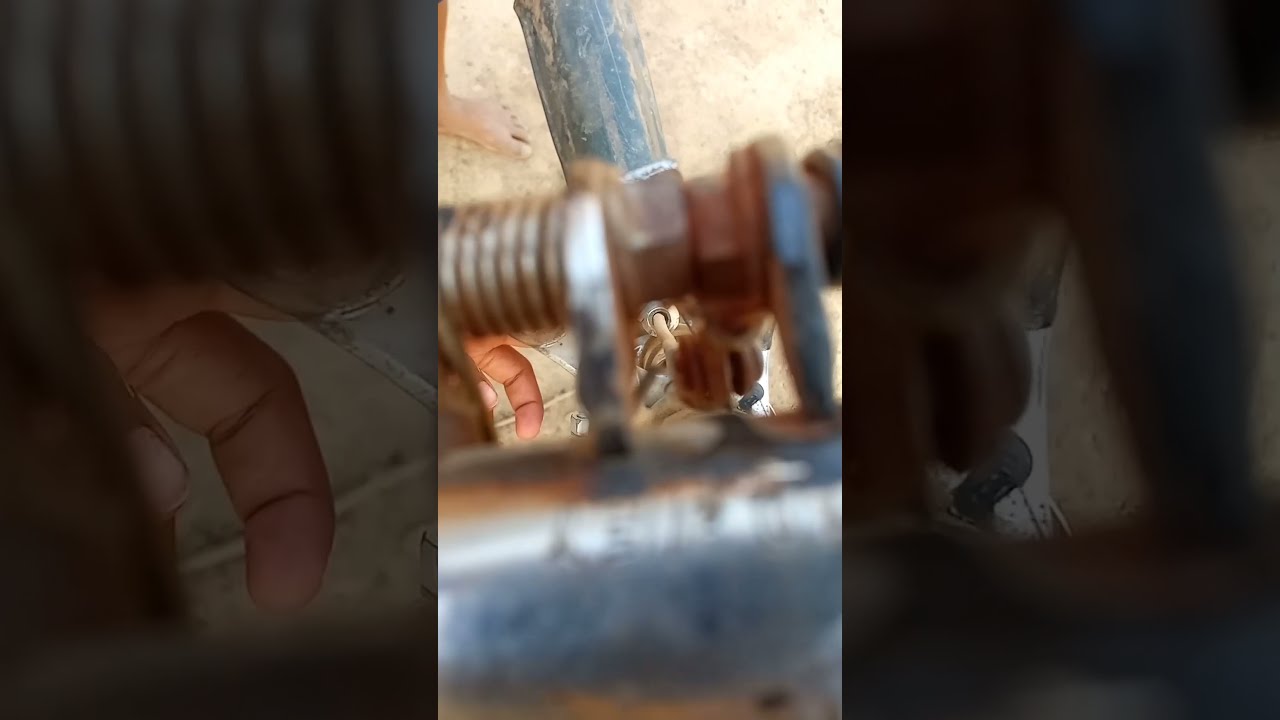This image is an extreme close-up depicting a section of a machine or piece of equipment, possibly a bicycle or motorcycle. Dominating the frame is a rusted silver metal pipe oriented vertically, with visible discoloration on its surface. Attached to this pipe are two fasteners, each incorporating a spring mechanism secured by nuts and bolts. In the background, another metal pipe runs perpendicularly, partially visible with a white tube inside. The out-of-focus foreground suggests a repair is underway, as evidenced by the partial view of brown-skinned fingers positioned beneath the components, indicating someone's hand at work. The surroundings show a dark tan ground, and the top left corner reveals what seems to be part of someone's foot, providing context that the scene is likely an outdoor setting.